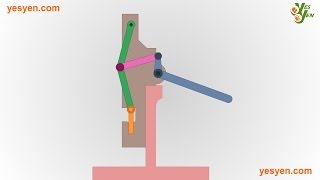The image showcases an object comprised of various geometric shapes against a light gray background, with the text "YesYen.com" prominently displayed in the upper left and lower right corners. In the upper right corner, there is a green logo of the same name. The central object appears to be an abstract or modern art piece, primarily depicted in a darkish brown color with interconnected lines and shapes in green, pink, yellow, and blue. A notable feature is a pink horizontal base with a connected vertical stick at its center, resembling an upside-down capital T. Additionally, green lines stem from the pink base, with a pink line connected to their middle, a yellow line at the bottom end, and a blue line branching out to the lower right and ending with another short blue segment. The entire composition presents a complex and abstract diagram that might symbolize some machinery or conceptual art, enhanced by colorful parts and connecting elements.